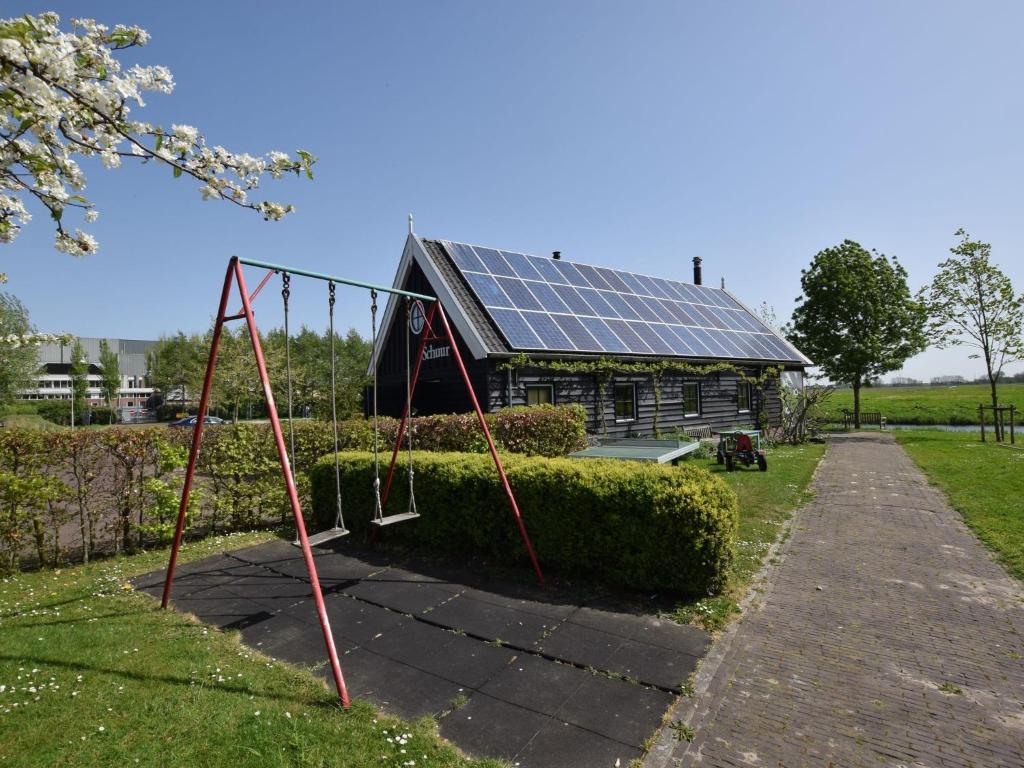In this brightly lit, daytime photograph, the landscape is dominated by lush, green grass and a brilliant blue, cloudless sky. Central to the scene, a cobblestone path winds through the middle ground, bordered by green, lush hedges and leading towards an old structure, possibly a house or recreational building, adorned with solar panels on its roof. The building, partially covered in creeping vines, features the faint lettering of "Schumer" on its front, indicating its historical significance. In the left foreground, a swing set with two swings, fashioned from steel or aluminum and painted red with chipped spots, stands on a black rubber padded area. The flat terrain extends towards a parking lot on the left, where a car is visible. Beyond, the landscape is adorned with more shrubbery and trees, including a prominent white flowering tree, adding to the tranquil and serene atmosphere of this potential historical site or peaceful recreational area.